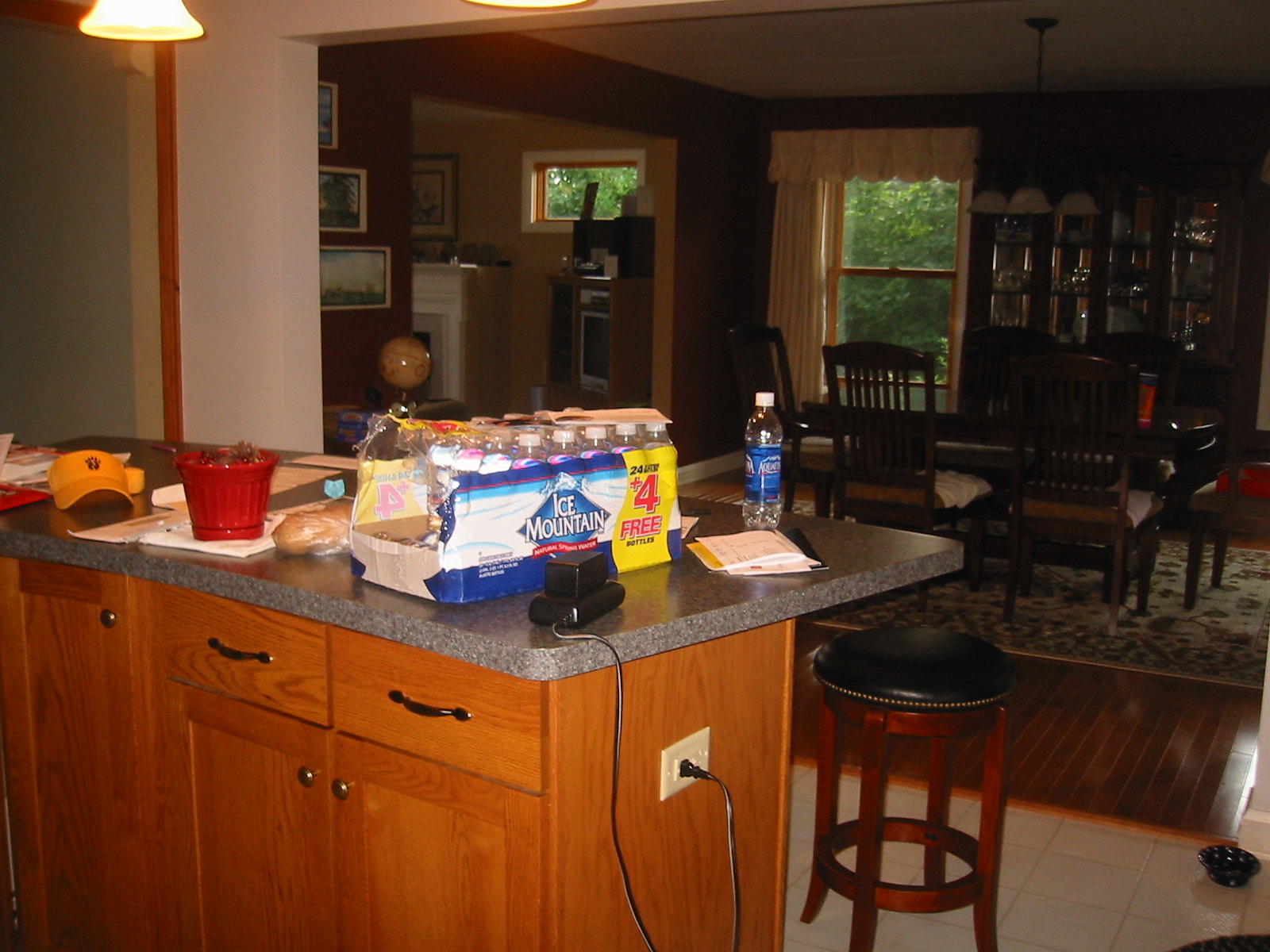In this photo, the foreground features a kitchen counter adorned with a variety of items. The counter, made of gray granite, is surrounded by a set of honey-brown stained wooden cabinets and drawers. At the far end of the counter, a black electronic device is plugged into an outlet. Adjacent to this device is a partially full bottle of water and an opened case of Ice Mountain water bottles. A stack of folded papers, likely the daily mail, rests on the counter next to a loaf of bread wrapped in clear plastic. Nearby, a red ceramic planter sits on a white towel, containing some dead or dying plant matter. A yellow baseball cap is also placed on the counter, which has a black leather stool with a dark wooden frame pulled up to it. 

The kitchen floor is tiled in white, while the adjoining dining room has a brown wooden floor. The dining room hosts a dark wooden rectangular table positioned over a cream and blue oriental rug. A window in the dining room is dressed with cream curtains, revealing a green tree close-up outside. In the distance, another room can be glimpsed, suggesting a spacious, interconnected living area.